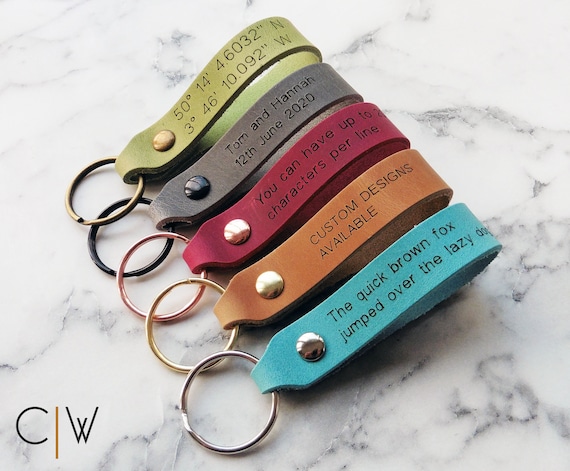The photograph captures a collection of five leather or faux leather keychain rings arranged on a white marble surface with grey striations. The keychains feature bands in various colors: pale green at the top, followed by dark grey, maroon, orange, and light blue towards the bottom. Each band is stamped with different text. The top green band displays a set of coordinates, while the dark grey band below reads "Tom and Hannah, 12th June 2020." The maroon band in the middle contains partial text about customizable characters. Below it, the orange band states, "custom designs available." Finally, the light blue band at the bottom features the phrase, "the quick brown fox jumped over the lazy dog." The bands are attached to rings in a variety of finishes, including gold, black, and silver. In the bottom left corner of the photo, an added black and orange logo reads "CNW."